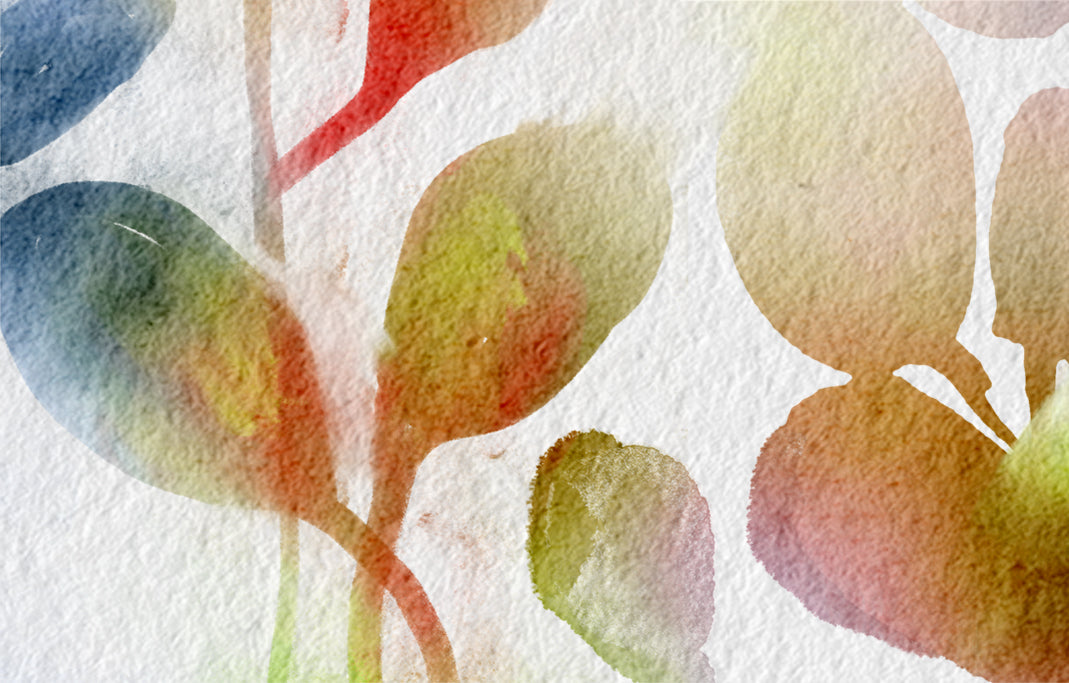The image depicts a wall adorned with a vivid painting of leaves and stems. The leaves, which are large and oar-shaped, are painted in a variety of colors including yellow, green, brown, white, red, and blue, standing out against a stark white background. At the center of the image, there's a prominent leaf with a stem extending downward, while another leaf with an upward-reaching stem is positioned to the left. In the upper left corner, a hint of a leaf can be seen, while on the far right, a cluster of three leaves with partial stems are depicted as silhouettes with minimal definition. The leaves’ outlines are clear, but they lack intricate details, allowing their bold colors to dominate the scene.